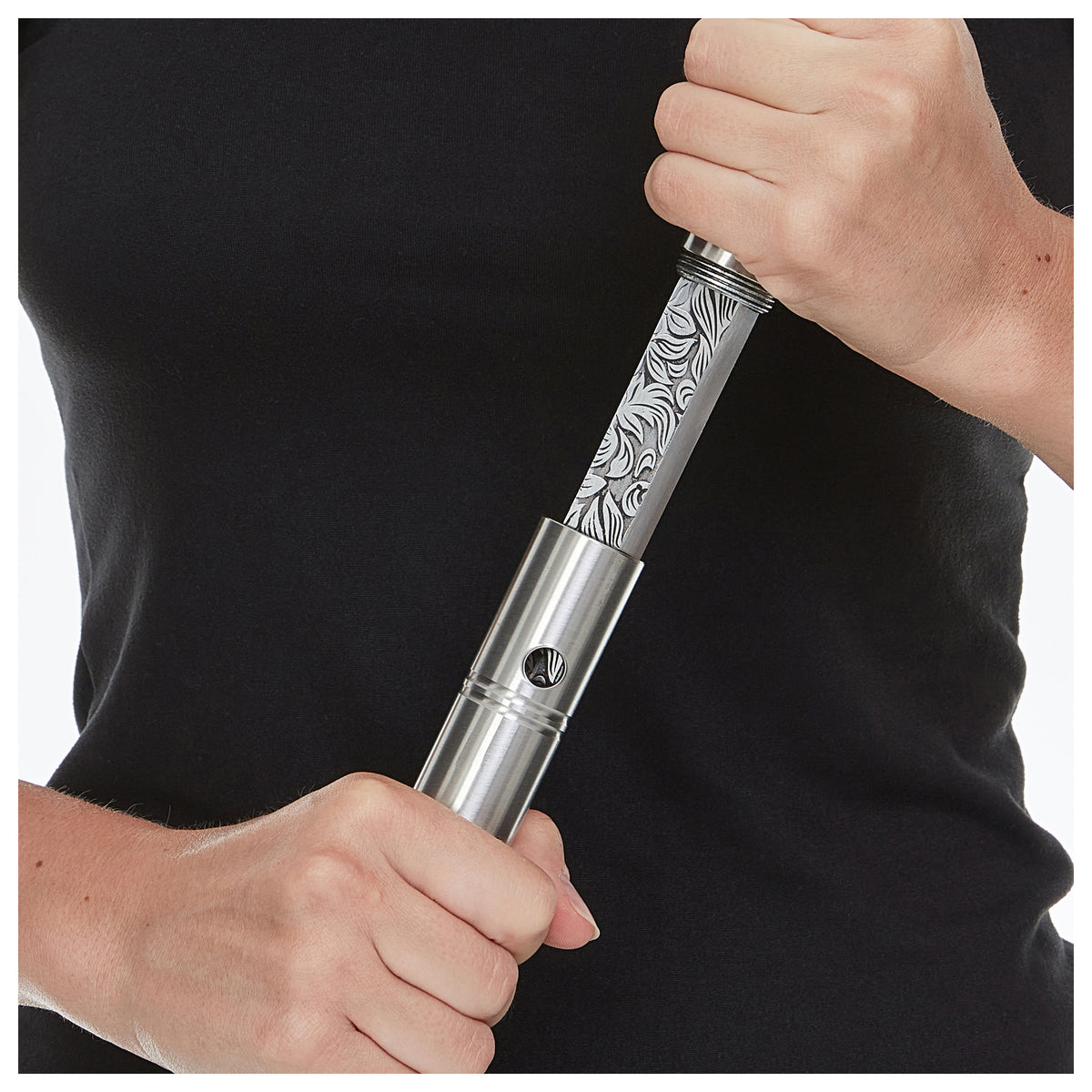This close-up photograph showcases the torso of a person of undetermined gender, wearing a black shirt. The individual is holding a sophisticated knife in their hands. The left hand is positioned at the top, gripping the handle of the knife and pulling it upward. Meanwhile, the right hand is lower, securely holding the scabbard, which appears to be made of polished silver metal. The knife itself is adorned with intricate leaf filigree patterns etched into the blade, suggesting it is a high-quality, possibly expensive piece. The sheath, also elaborate, features a small hole near the top and double lines carved just below this opening, potentially serving as a locking mechanism to secure the knife when sheathed. The background of the image is a plain white, ensuring all focus remains on the knife and the hands holding it.